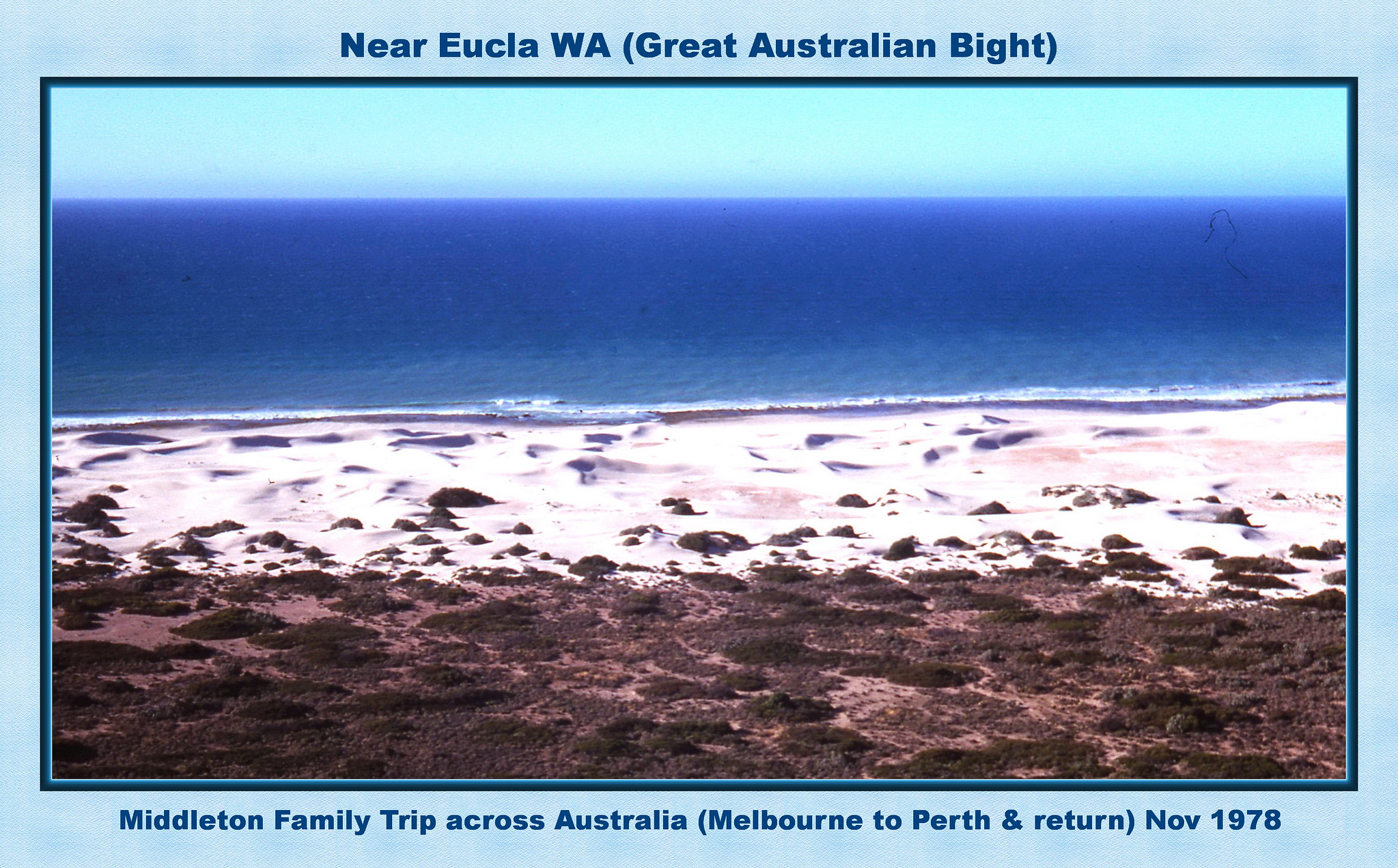The image features a personal photograph bordered in light blue with the following text in capital letters along the top: "Near EUCLA WA (Great Australian Bight)." Along the bottom, the text reads: "Middleton family trip across Australia (Melbourne to Perth and return) November 1978." The top half of the image shows a brilliantly blue sea meeting a teal or light blue sky, with the horizon cutting across the midsection. The sea displays small white caps near the shore. Below, the coastline features very light tan, almost white sand with small dunes, transitioning to a foreground with patches of green grassy areas interspersed with brown soil. The overall colors in the photograph include light blue, dark blue, white, tan, green, and brown, adding to the detailed depiction of a beach scene taken during a family trip in late 1978.